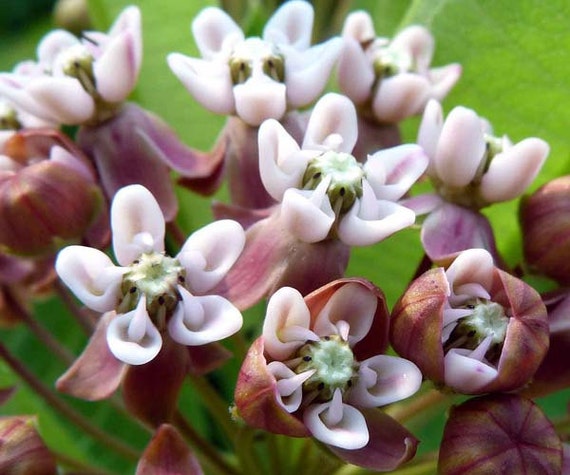The image captures a vibrant, green, grassy background that sets the stage for the main focus: several stunning, light pink flowers in full bloom. Each blossom boasts five thick petals with delicate holes near the center, which reveals a light green middle adorned with spindly filaments. The outer shell of the flowers is a distinctive purpley-red, almost burgundy, adding depth and contrast to the composition. The stems display a mix of burgundy and green hues, further enriching the visual tapestry. In the foreground, some flowers stand prominently, while others are more muted in the background. The overall scene exudes a sense of natural beauty and vivid detail, capturing at least nine of these healthy, blooming flowers.